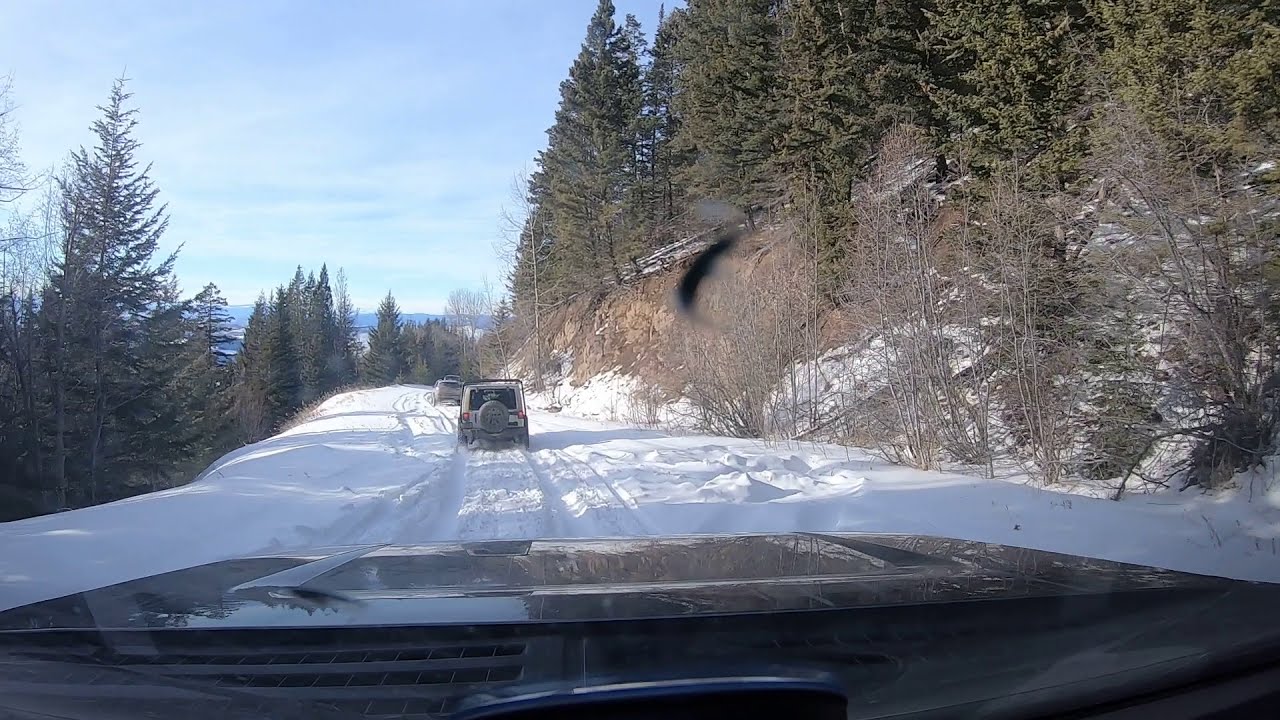This image captures a snowy, mountainous road scene from the perspective of a black SUV, possibly part of a convoy. The road, completely blanketed in snow, shows tire tracks from numerous vehicles. In front of the viewer, there are at least two vehicles—a Jeep with a tire mounted on its rear and another SUV or pickup truck. To the left of the road, a dense array of tall pine trees lines a slope, while to the right, a hill also adorned with evergreens and some bare trees rises upward. The daytime sky overhead is a beautiful blue, scattered with wispy, hazy clouds, indicating a clear, yet cold, winter day. The scene is picturesque yet suggests a cautious drive through the snowy, possibly treacherous, mountain pass.